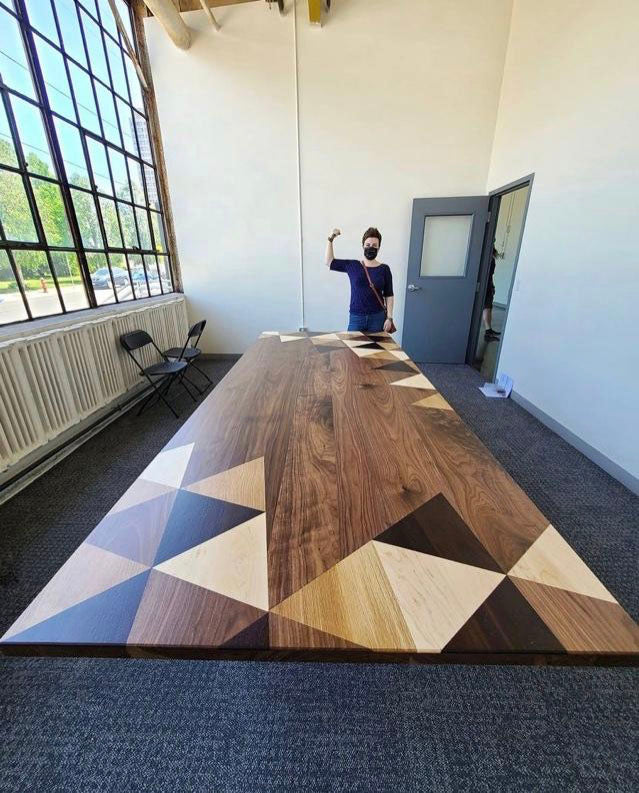The photograph shows a narrow room with white walls and a dark blue, grayish-blue carpet. On the left side of the room, there is a large, many-paned window that offers a view of a blue sky, some trees, and a few cars outside, indicating daytime. Below the windows are radiator or air circulation vents. In the center of the room stands an exquisite long brown wooden table, with triangular patterns in varying shades of brown at each corner. The table spans from the background near the open blue door with a window, up to the foreground. 

On the left side of the table, there are two black folding chairs facing opposite directions—one towards the door and the other towards the window. At the far end of the table is a woman wearing a blue shirt, jeans, a tan purse slung over her shoulder, and a black face mask. She is striking a muscle pose with her left arm raised and fist closed. Near the open door on the right-hand side of the room, papers are scattered on the floor, and a person's leg clad in a black shoe is visible, suggesting someone is entering the room.